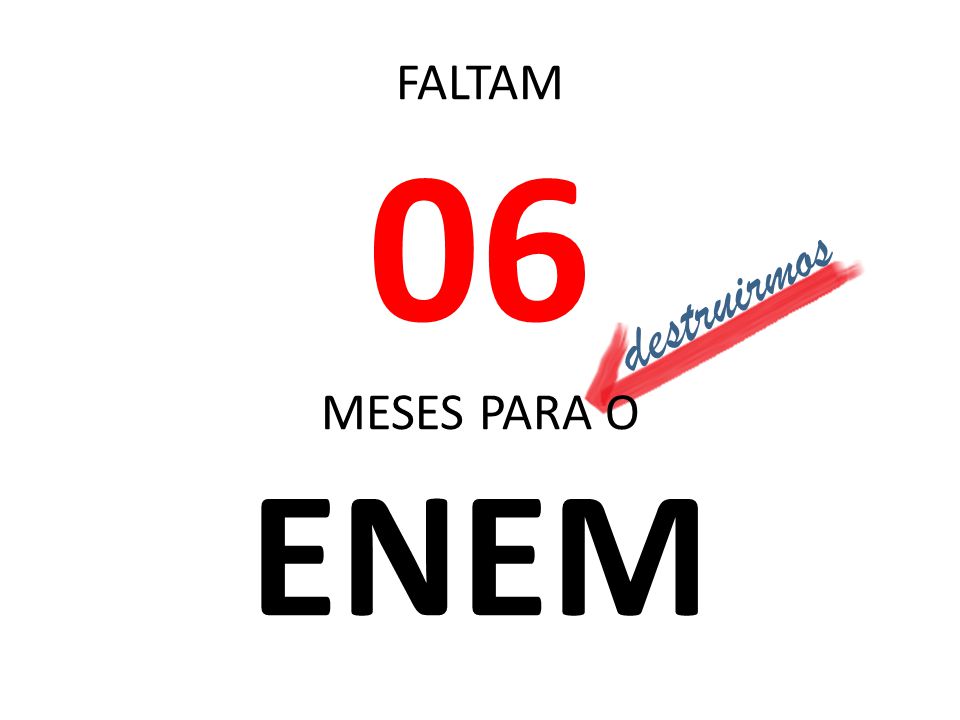The image features a plain white background dominated by a series of texts in varying styles and colors. At the very top, in all capital black letters, it reads "FALTAM." Directly below, in a much larger red font, is the number "06." Underneath this, again in capital black letters, is the phrase "MESSI'S PARA O." A red arrow points towards the word "PARO," adding emphasis. Additionally, in a diagonal slant and dark blue cursive letters, the word "DESTRUIRMOS" appears across the image. At the very bottom, in very large, bold black letters, is the word "ENEM." This configuration of variously colored and styled text elements forms a striking visual on an otherwise empty white canvas, creating a message that's meant to stand out.